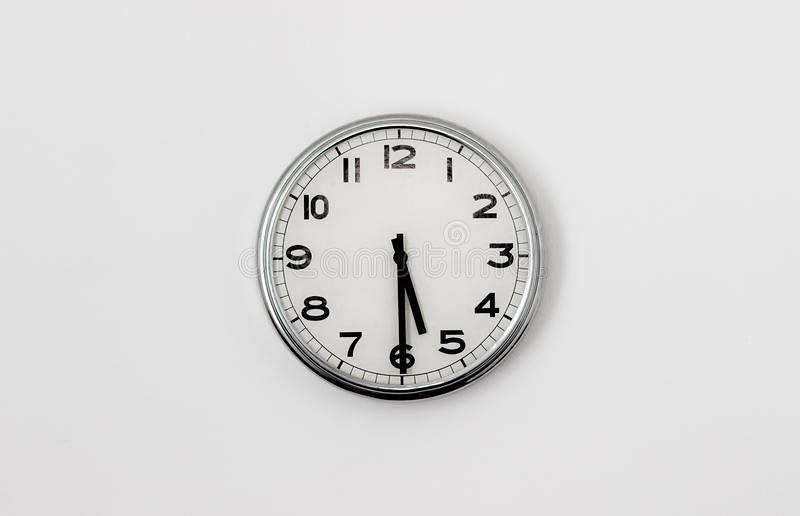The image depicts a white round clock mounted centrally on a solid white wall, which is slightly rectangular, being wider than it is tall. The clock is accentuated by a thin, silvery metallic border that encircles its face. Prominent black numbers marking the hours encircle the clock’s face, with the black hour and minute hands indicating a time of approximately 5:30. Between the numbers and the outer metallic border is a series of fine black lines, each denoting a second, with bolder lines marking the positions of the main numerals (1, 2, 3, etc.), enhancing the clock's classic design.